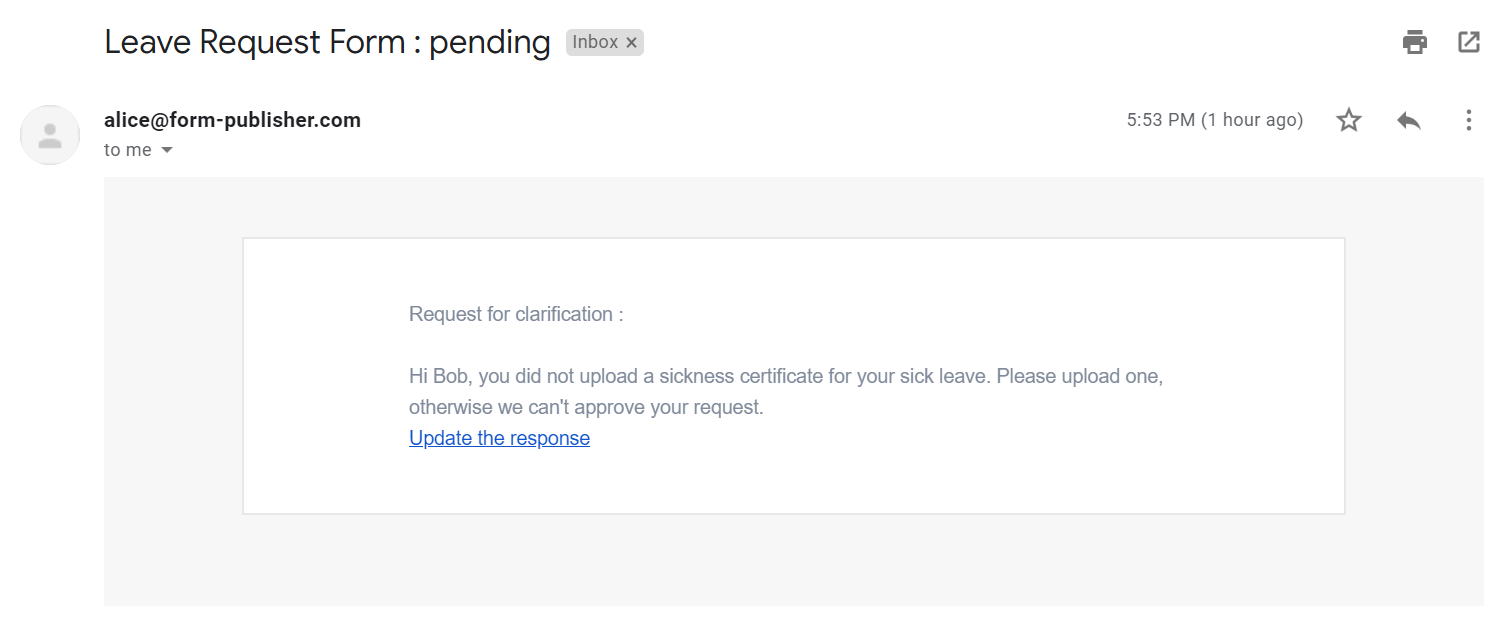The image depicts an email from Alice at formpublisher.com to Bob, addressing a pending leave request. The email subject is "Request for Clarification," and it highlights the need for Bob to upload a sickness certificate for his sick leave to get the request approved. The message is straightforward: 

"Hi Bob, you did not upload a sickness certificate for your sick leave. Please upload one. Otherwise, we can't approve your request."

A blue hyperlink labeled "Update the Response" is available for Bob to click on and provide the necessary documentation. The email was sent by Alice at 5:53 p.m., with the timestamp indicating "an hour ago." Alice’s profile image is a generic, computer-generated avatar.

At the top of the email interface, several icons allow Bob to print the email, mark it as a favorite, reply, and adjust the email window size. Additionally, there are three dots that offer a menu with more options when clicked. The overall layout is clean and user-friendly, making it easy for Bob to understand and act on the request.